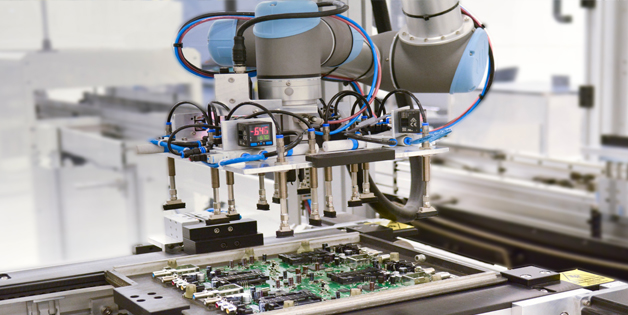In this brightly lit photograph taken inside a pristine white factory or research center, a large, intricate machine dominates the scene. The facility features two assembly lines converging from the bottom left to the top left and right of the image. Central to the machinery is an expansive circuit board, primarily green with an array of black components including transistors, capacitors, and integrated circuits. This circuit board, potentially part of a larger motherboard, is adorned with numerous knobs and metal parts. Above, an automated mechanism, festooned with blue and red wires, is in the process of meticulously assembling or attaching additional components to the circuit board. Prominently visible are a pressure gauge and a digital display panel glowing with the number -645 in red font, indicating the precise conditions under which the machinery operates.